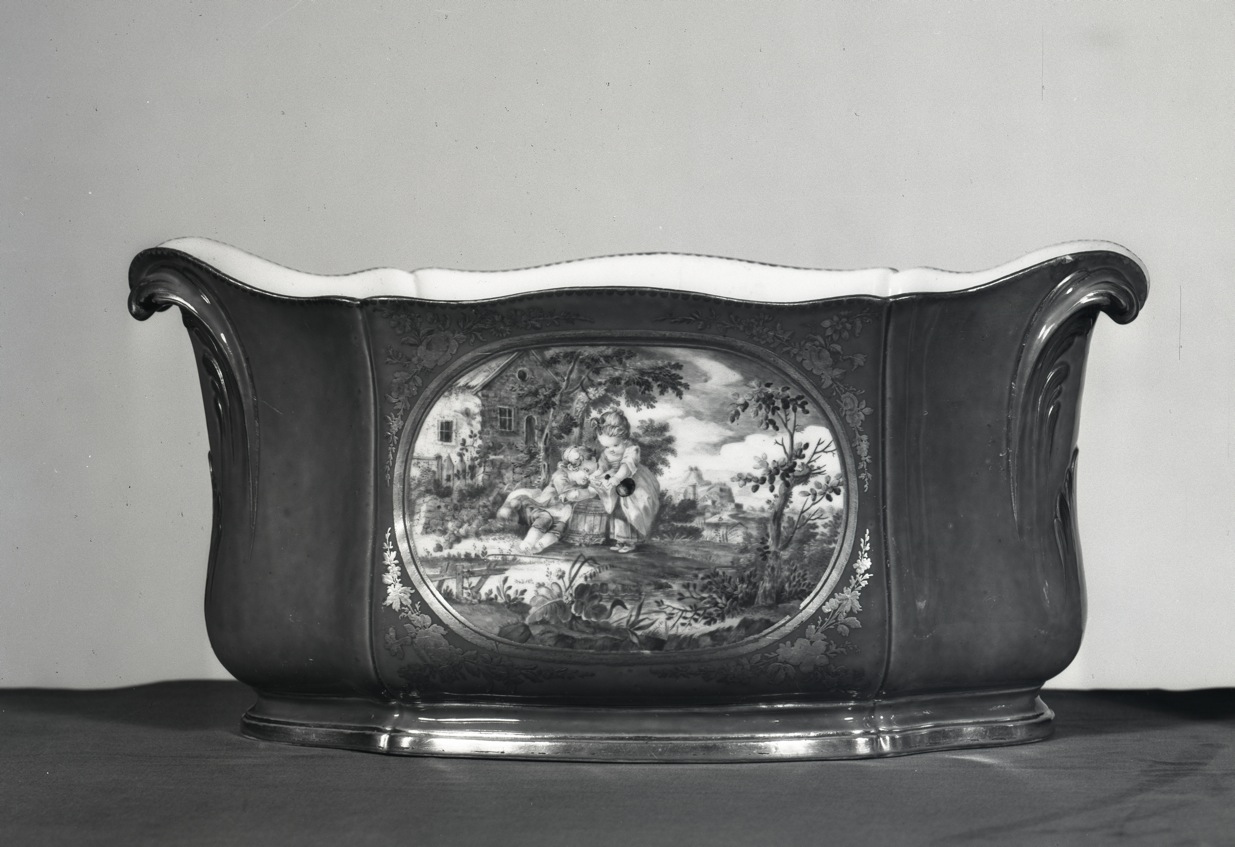This is a detailed black and white photograph of a horizontal, dark-colored ceramic dish with a white interior. The dish features an intricate design along its sides, ornamental waves pointing outward, and a small, circular base with an indentation. It sits atop a dark fabric against a white wall backdrop. Central to the front face of the dish is an oval-shaped illustration bordered by floral patterns. Inside the oval, the scene depicts two children dressed in white, engaged with an object, possibly a barrel, in front of a stone-walled house featuring a pitched roof and several windows. The house is situated amid plants, trees, and other building-like shapes under a dark sky with white clouds. The children, a young girl appearing to console a small boy, resemble figures of European descent in aristocratic early 50s attire. The dish's exterior also suggests a reflective, shiny silver bottom.